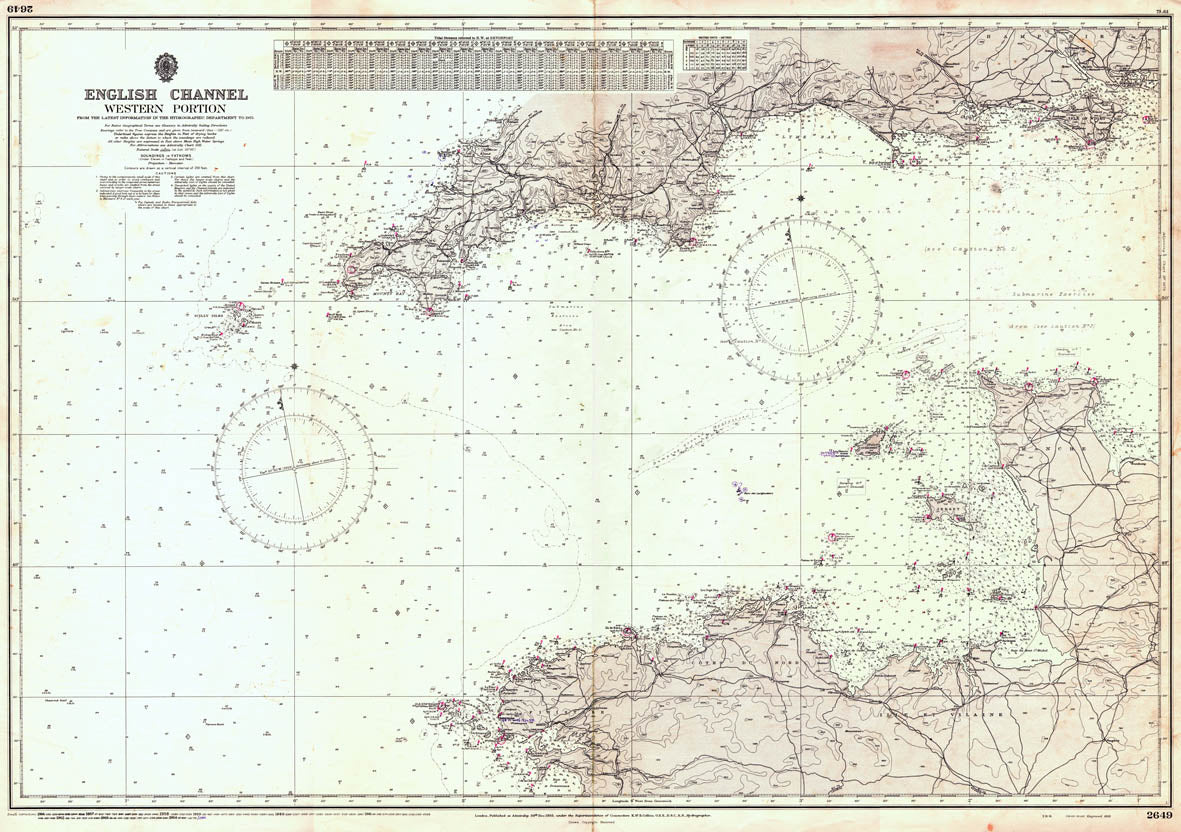This image is a detailed, yet somewhat aged, nautical map of the Western portion of the English Channel. The map's predominant background color is a cream shade with light tan and brown markings, and a pale pink hue for landmasses. The title "English Channel, Western Portion" is prominently displayed at the upper left corner, accompanied by smaller, unreadable text likely containing copyright information and technical specifics. 

The map delineates the coastlines of both southern England at the top and northern France at the bottom, highlighting varied and intricate landforms. Major roads and towns along these coastlines are also depicted, although the fine print is not legible. There is a legend or infographic at the top center of the map, providing context to the symbols, albeit unreadable. 

A notable feature includes two compass-like symbols centered in the water area, characterized by double wheels with crossing lines. Additionally, ruler markings frame the entire map. Various dots scattered across the water likely represent navigational aids or measurement devices. The map's texture and color palette suggest it originates from a period between the Victorian era and the early 20th century, although no specific date is visible.